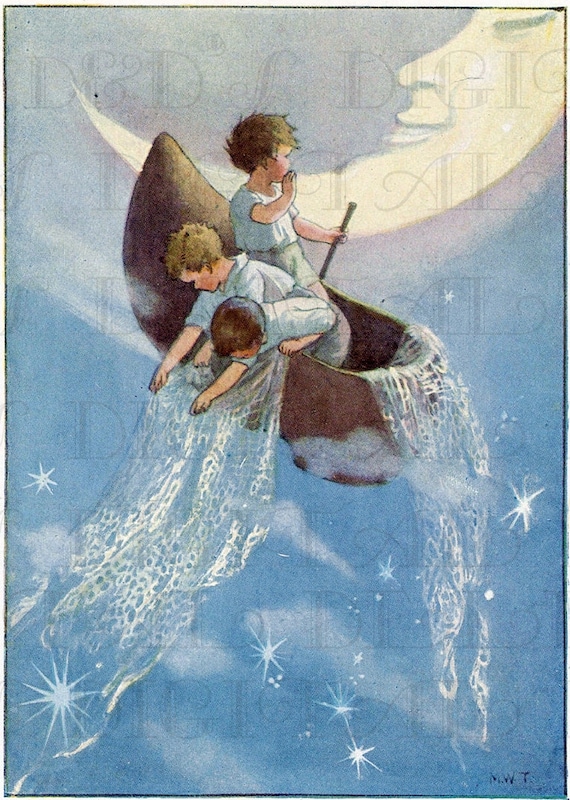A detailed drawing depicts three young boys in a canoe-like boat floating against a surreal, light blue backdrop that suggests they may be canoeing through the sky. At the top of the image, a crescent moon with a human-like face, complete with eyes, a nose, and a mouth, watches over them. One of the boys, with dark hair, faces away from the viewer and holds an oar while gesturing towards the moon as if whispering to it. The other two boys, one with brownish-blonde hair and the other with dark blonde or brown hair, lean over the side of the boat closest to the viewer. They are seen pulling in a shimmering, insubstantial net made of white and silver material, which glistens like gossamer threads. Both boys wear bluish shirts and grayish pants. The ambiguous setting, with stars and clouds visible and the net-like material resembling water, creates an ethereal scene that blurs the lines between sky and water. The overall style of the drawing suggests it could be an illustration from an old book or a vintage painting. A faint watermark with the letters "D," "A," and "L" runs vertically behind the illustration.